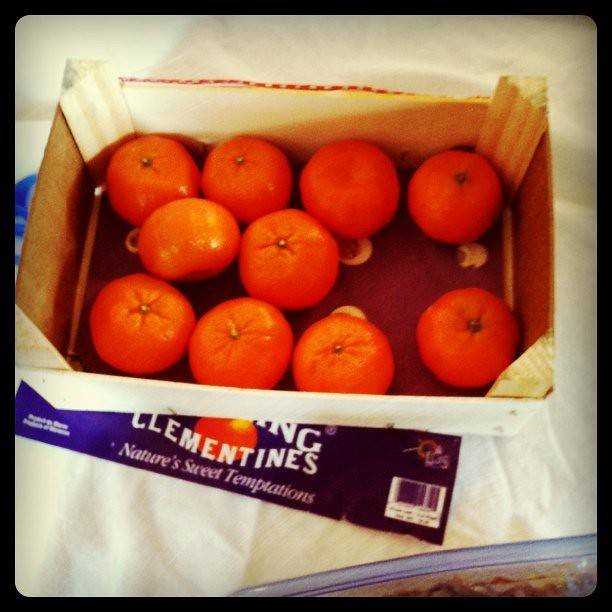This photograph features a white cardboard box with eight to ten clementines, or "cuties," nestled inside. The box is constructed with simple pine slats on the sides and supported by four angled wooden posts at the corners. A piece of die-cut paper or cardboard, showing slight rumples and textures, lines the bottom. The arrangement of the fruits includes four clementines at the front edge, four at the back edge, and two in the middle. A partially visible printed label on the side of the box, adorned in purple or blue, reveals a logo of a clementine and a tagline reading, "Clementines, Nature's Sweet Temptation." Additional features include a barcode and an obscured brand name ending in "ING." The setting includes a white surface that might be a tablecloth, and the image edges are darkened, possibly indicating a filter. A blurred, indeterminate object, which could be a crumpled Ziploc bag with a brown substance inside, lies near the box.